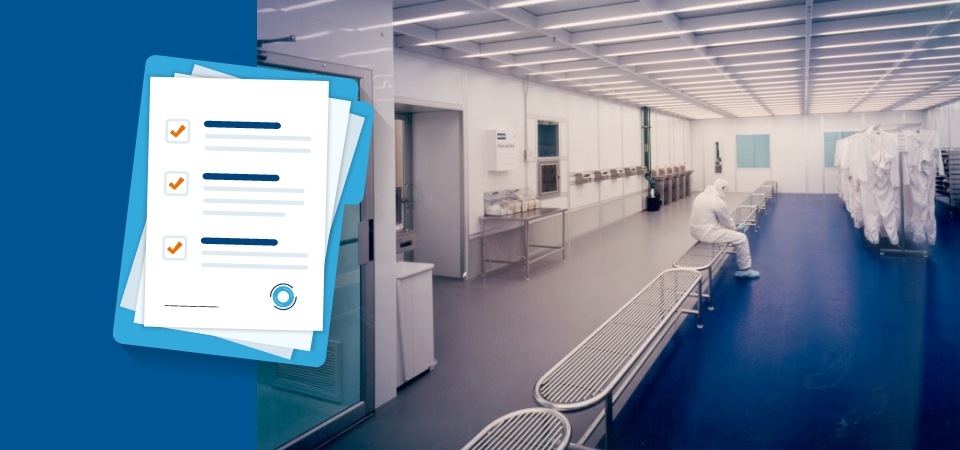The image depicts the interior of a medical laboratory, characterized by a distinctive blue and tan flooring that transitions across the scene. In the foreground, seated on one of a series of metal benches that extend towards the right, is a man dressed entirely in white, reminiscent of a decontamination or hazmat suit. His attire includes blue plastic wraps over his shoes, emphasizing cleanliness and contamination control. The man appears contemplative, with his head bowed. Centrally located to his right is a movable rack filled with identical white uniforms, ready for use. The background features a series of sinks and blow dryers, complemented by white bins intended for disposable items, such as plastic gloves. Near these utilities is an open doorway to the left. A notable digital embellishment on the image includes a clip art depiction of a bright blue folder, containing white papers marked with orange check marks, though this is clearly not part of the actual laboratory environment.